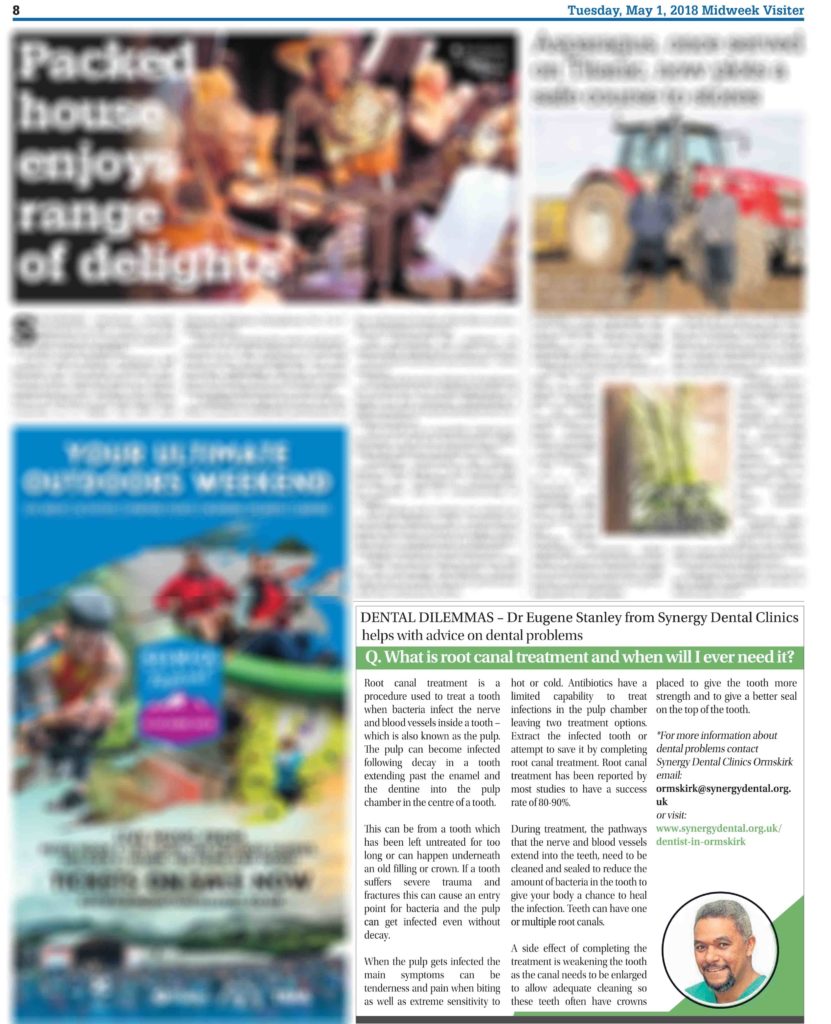The image depicts a news webpage with the top articles blurred, making only the bottom right corner article visible. The article is titled "Dental Dilemmas" and features advice from Dr. Eugene Stanley of Synergy Dental Clinics on various dental issues. A green bar runs horizontally across the segment, containing text in white font that begins with "Q." followed by the question, "What is root canal treatment and when will I ever need one?" Below this, the response begins, explaining that root canal treatment is a procedure used to address a tooth infection when bacteria infect the nerve and blood vessels, known as the pulp. The detailed answer spans three lines. Accompanying the text is an image of Dr. Eugene Stanley in the lower right-hand corner.